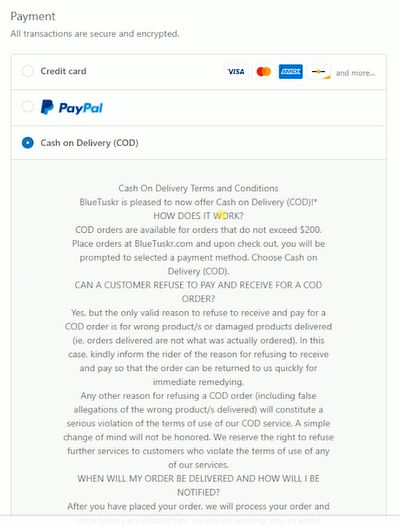Screenshot Overview of Blue Tusker Payment Option with Cash on Delivery (COD) Terms and Conditions

This screenshot captures the payment section of an online checkout process. At the top, bold text reads "Payment," reassuring potential customers that all transactions are secure and encrypted. Several payment methods are listed, including Credit Card (Visa, MasterCard, Amex, and more), PayPal, and Cash on Delivery (COD). The COD option has been selected.

Highlighted beneath is a detailed description of Blue Tusker's Cash on Delivery (COD) service, formatted with guidelines and conditions. The text begins with an introduction: "Blue Tusker (spelled capital B-L-U-E, capital T-U-S-K-R) is pleased to now offer cash on delivery (COD)."

A section titled "How does it work?" explains that COD orders are available for purchases not exceeding $200. Customers are instructed to place their orders at bluetusker.com, where they will be prompted to select a payment method during checkout. The "Cash on Delivery (COD)" option should be chosen.

The next section addresses a frequent concern: "Can a customer refuse to pay and receive a COD order?" The policy allows customers to refuse COD orders only if incorrect or damaged products are delivered, clearly explained as orders that are not what was actually ordered. In such cases, customers should inform the courier of the refusal reason so the order can be quickly returned and corrected. Refusing an order for any other reason, including false claims of wrong products, is considered a serious violation of the COD service terms. A simple change of mind does not qualify, and customers who violate these terms may be denied further services.

The final visible section answers the question, "When will my order be delivered and how will I be notified?" It states that once an order is placed, it will be processed, but the rest of the text is cut off at the bottom of the image, leaving the full details incomplete.

This comprehensive explanation of Blue Tusker's COD service aims to ensure customers understand the terms and conditions, promoting transparency and proper use of the service.